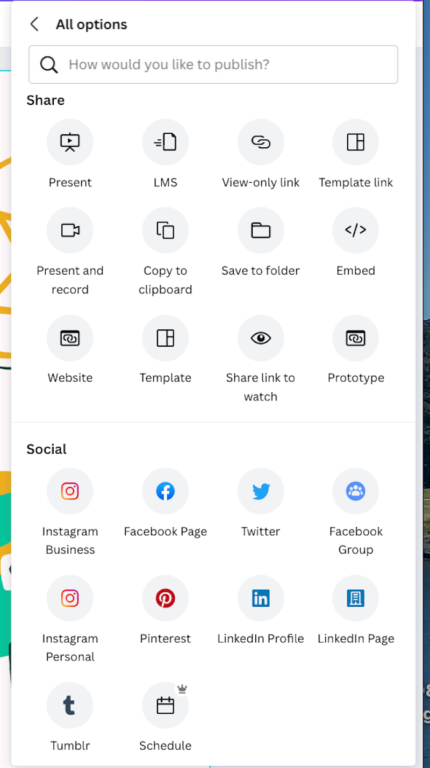This image showcases a comprehensive interface featuring a variety of icons and options for sharing and publishing content. At the top, there is a navigation bar that includes a back arrow and a search field adorned with a magnifying glass icon along with the prompt, "How would you like to publish?". Below this, there is a section dedicated to sharing options, each represented by distinct icons:

- **Present**: Depicted with a screen and a play button.
- **LMS**: Illustrated with a file icon.
- **View Only Link**: Represented by interconnected paper clips.
- **Template Link**: Symbolized with a square icon.
- **Present and Record**: Displayed with a camera icon.
- **Copy to Clipboard**: Featuring an image of a clipboard.
- **Save to Folder**: Embellished with a folder icon.
- **Embedded**: Illustrated by two arrows pointing away from each other with a slash.
- **Website Button**, **Template**, **Share Link to Watch**, and **Prototype**.

Additionally, under the **Social** section, users can find icons for various social media platforms and functionalities:

- **Instagram Business**: Featuring the Instagram logo.
- **Facebook Page**: Emblematic with a blue 'F' icon.
- **Twitter**: Identified by a blue bird icon.
- **Facebook Group**: Depicted with a lighter blue icon showcasing a group of people.
- **Instagram Personal**: Displayed with the Instagram logo.
- **Pinterest**: Characterized by a white 'P' on a red background.
- **LinkedIn**: Marked by an 'IN' icon.
- **LinkedIn Page**: Similar to the LinkedIn icon.
- **Tumblr**: Presented with a 'T' icon.
- **Schedule**: Illustrated with a calendar symbol.

The entire interface is set against a clean white background with black text, ensuring clarity and ease of use for navigating through the varied sharing and publishing options.